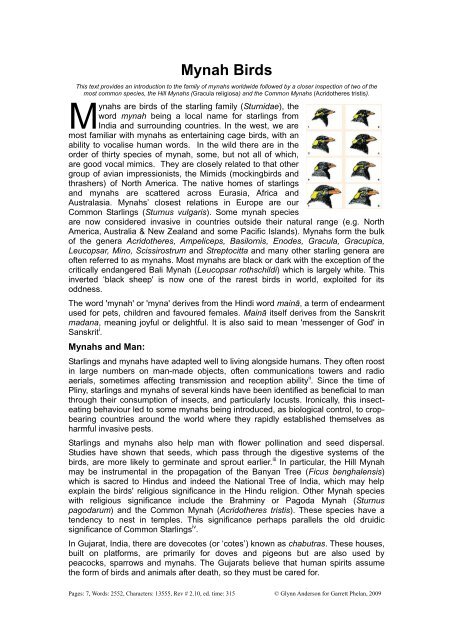The image depicts a black-and-white newspaper or magazine article titled "Myna Birds," prominently displayed in bold at the top. Below the title is a two-line italicized blurb, followed by about six paragraphs of descriptive text explaining the history and characteristics of Myna birds. The initial letter "M" in the opening paragraph is accentuated in a larger, ornate font. The article starts by detailing that "Minas are birds of the starling family," highlighting their native name, origin from India, their ability to vocalize human words, and mentions approximately 30 species with varying mimicry skills. To the right of the text are eight illustrations organized in two columns and four rows, showcasing detailed drawings of Myna bird heads with distinctive black feathers and yellow markings on their necks. Further into the article, bold headers like "Minas and Man" segment additional information. The entire piece is set against a white background with crisp, black text for clear readability.